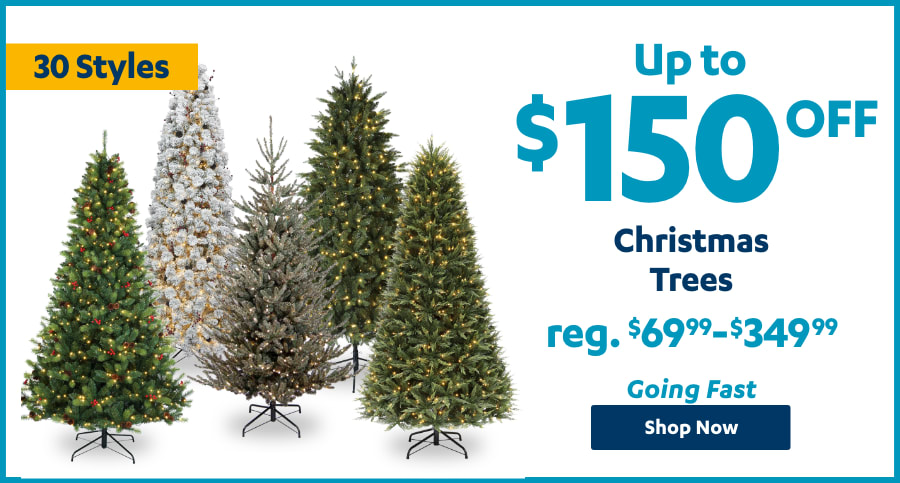This image is a promotional shopping page for Christmas trees, featuring a vibrant and festive design. It showcases four Christmas trees, one of which is white, while the others display varying shades of green, yellow, and blue. At the top left corner, there are 30 yellow stars adding a whimsical touch to the layout. The page advertises trees priced up to $150, previously listed between $699 and $349.99, with a note indicating they are selling quickly and encouraging customers to "Shop Now." The entire image is framed by a blue border, enhancing its visual appeal and making the promotional details stand out.